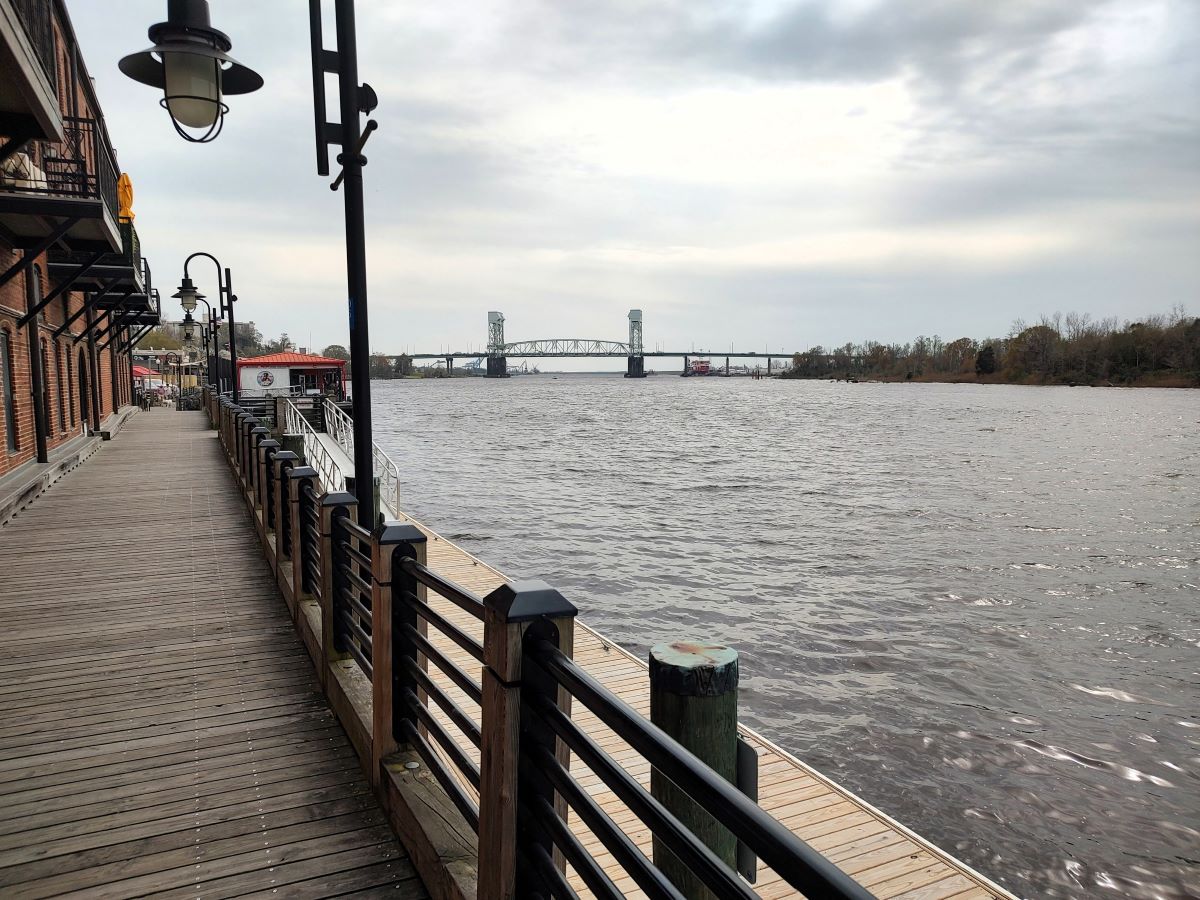This photograph captures a serene riverside scene as viewed from a boardwalk. On the left side of the image, the long façade of a brick building with black metal balconies on the second floor stretches into the frame. Below the building, the boardwalk is composed of gray horizontal strips of wood. Adjacent to this is a section with black metal pipes that run through robust wooden posts, adding an industrial touch. To the right of this segment, another lower boardwalk made of lighter-colored wood continues towards the river. The river itself has dark, reflective water beneath a gray, overcast sky. A metal bridge, with two prominent towers at each end and a slight arch in the center, spans the river horizontally a little above the center of the photo. On the right bank of the river, a thin line of brown, low bushes marks the boundary between land and water, adding to the natural yet subdued palette of the scene.